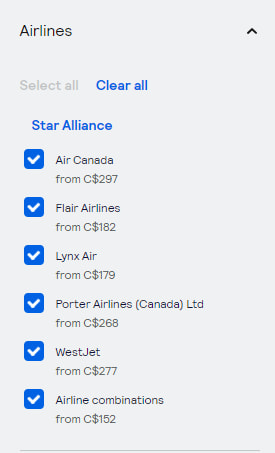This image captures a detailed screenshot of a person comparing various airline flight options for a trip to the same destination, meticulously organized in a list format from top to bottom. The header of the screenshot reads "Airlines," followed by a comprehensive breakdown of options available through different carriers. The list includes:

- Star Alliance, Air Canada with prices starting from $297
- Flair Airlines from $182
- Lynx Air from $179
- Porter Airlines Canada Limited from $268
- WestJet from $277
- Airline Combinations from $152.

The screenshot highlights the substantial variation in ticket prices among the airlines, suggesting an effort to find the best value for money. Subtle details and the structured format of the list demonstrate the user's attempt at a comparative analysis to determine the most economical flight choice.